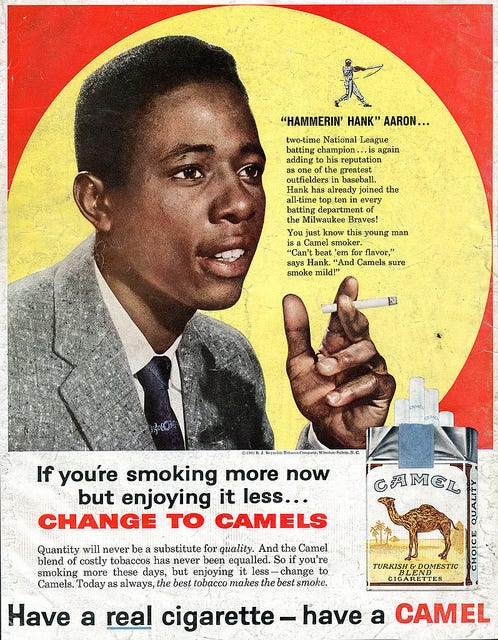This is a vintage magazine advertisement for Camel Cigarettes featuring the legendary baseball player, Hank Aaron. Set against a vibrant red background with a central yellow circle, this ad prominently displays a nostalgic image of Hank Aaron, either a photograph or an artful rendering, dressed in a suit and tie while holding a cigarette, looking off to the right. Above him is an illustrated depiction of Aaron swinging a baseball bat. A headline introduces him as "'Hammerin' Hank Aaron," emphasizing his accolades as a two-time National League batting champion and one of the greatest outfielders.

The text next to his face states, "Hammerin' Hank Aaron, two-time National League batting champion, is again adding to his reputation as one of the greatest outfielders in baseball. Hank has already joined the all-time top ten in every batting department of the Milwaukee Braves. 'You just know this young man is a Camel smoker. Can't beat him for flavor,' says Hank, 'and Camel sure smokes mild.'"

Below this narrative, the main call-to-action reads, "If you're smoking more now but enjoying it less, change to Camel's." It further elaborates, "Quantity will never be a substitute for quality, and the Camel blend of costly tobaccos has never been equaled. So if you're smoking more these days, but enjoying it less, change to Camel's. Today, as always, the best tobacco makes the best smoke."

To the right side of the ad, a detailed image of a Camel cigarette pack with four cigarettes peeking out stands prominently. Underneath, it concludes with the tagline, "Have a real cigarette. Have a Camel." The striking red and yellow color scheme, along with the classic layout and vintage imagery, make this ad a nostalgic tribute to both Hank Aaron and the era it represents.